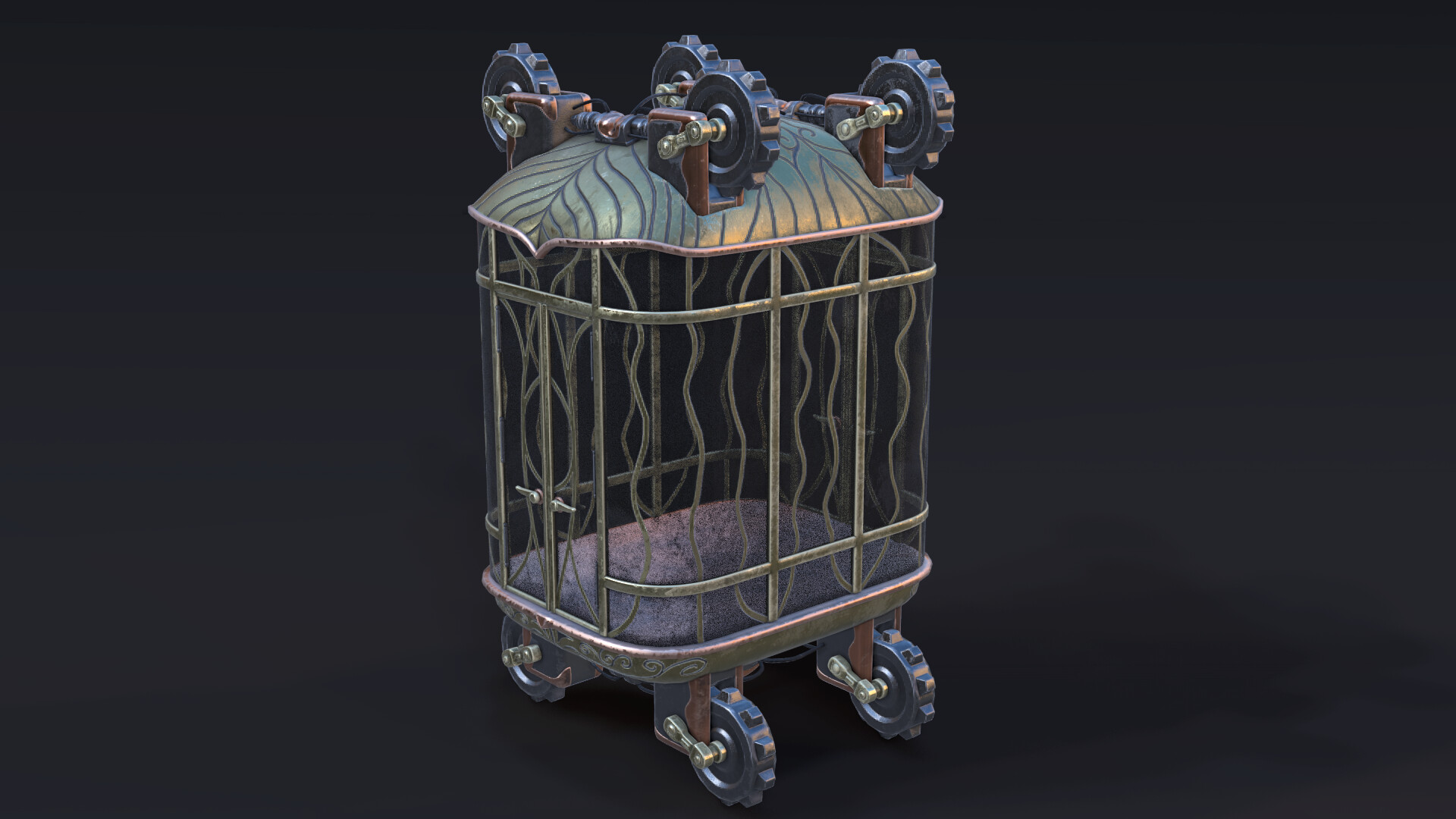The image is a detailed and intricate piece of digital art portraying a 3D object that resembles an old-style elevator or a cage-like structure. This object is set against a completely black background, enhancing its striking features. 

The base of the structure is a square with rounded edges, bordered by a decorative, gold-colored trim. Rising from the base are clear walls, reinforced with golden metal bars that form a loopy, decorative pattern. These bars add an ornate touch to the structure, hinting at a bygone era. At the very top, there is a shell-like metal component, also bearing intricate patterns etched into it, and a brassy gold hue that complements the bars.

Interestingly, the structure is equipped with wheels—four on the top and four on the bottom. These wheels have a dark gray color with notches or grooves, resembling gears. These gear-like wheels add an industrial feel to the otherwise decorative piece. Additionally, a small door is noticeable on one side of the structure, suggesting it could potentially house a small animal. A close examination reveals a lock near the wheels, indicating that the bottom part can be secured, possibly to prevent movement or to lock the door. This amalgamation of ornate and functional elements creates a captivating and enigmatic object that bridges the past and the industrial age.